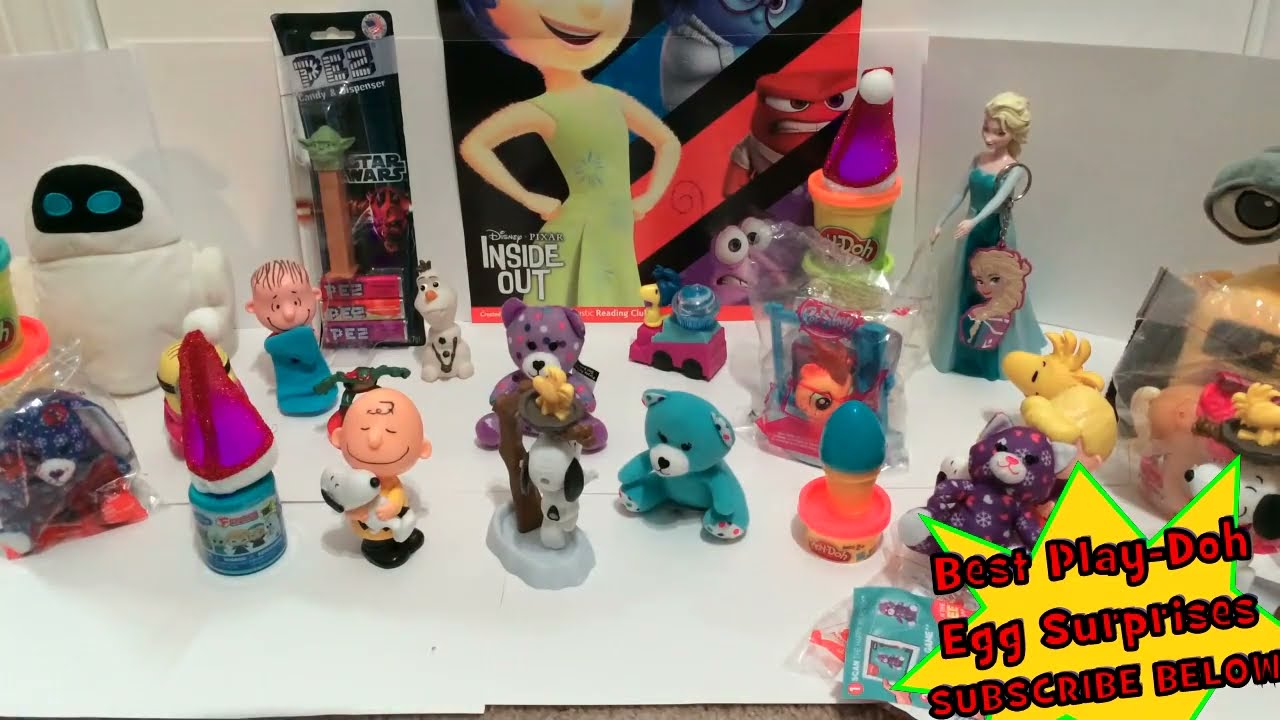The wide, rectangular image, taken from a slightly elevated angle, features an assortment of children's toys arranged on a white surface that appears to be made up of several stacked sheets of white paper. In the top left section, a Yoda PEZ dispenser is perched atop three PEZ packages, accompanied by a white robot stuffed animal. Nearby are several figurines from the Peanuts cartoon, including Charlie Brown and Snoopy. The back middle area showcases a poster for the Disney Pixar movie "Inside Out," with an array of Beanie Babies and stuffed animals, some of which are blue, teal, and navy blue adorned with daisy patterns, positioned in front. Additional figurines, including a gnome with a red triangular hat, populate the right side of the image along with other teddy bears, one of which is purple with black and red dots hugging a black and white bear. In the bottom right corner, a white and yellow star with green outlines features red text reading "Best Play-Doh Egg Surprises," with the instruction "Subscribe below" underneath.